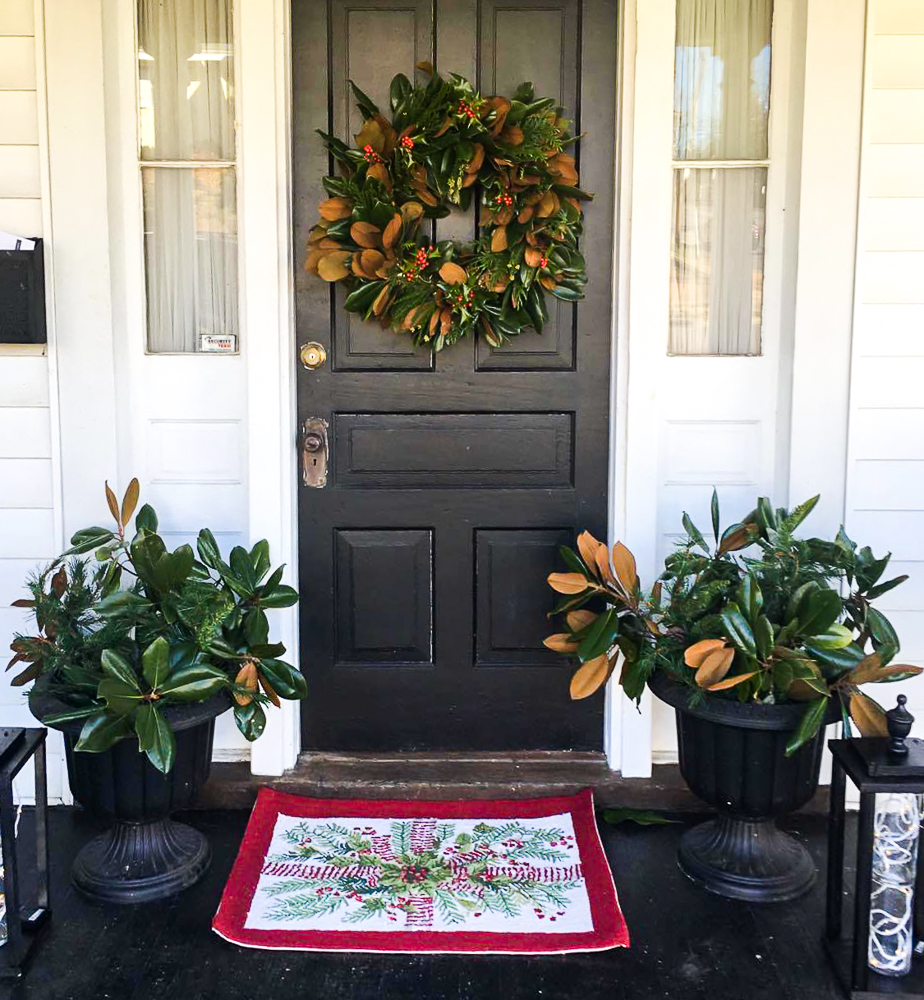This detailed photograph captures the elegant front entrance of a traditional white house, taken during the daytime. The focal point is a black front door, accentuated by a magnolia wreath with autumn colors and flanked by window panels, each covered by curtains. The entrance is framed by black, wooden steps leading up to a black deck. A white doormat with a violet-red border and a Christmas theme featuring poinsettia and pine branches warmly welcomes visitors. On either side of the door, there are large matching black planters containing lush, dark green leafy plants. In front of each planter stands a small, black rectangular lantern with a knob on top, adding a touch of charm to the setting. The house and its décor, including the hanging plant on the door, are in excellent condition, presenting a picturesque and inviting scene.